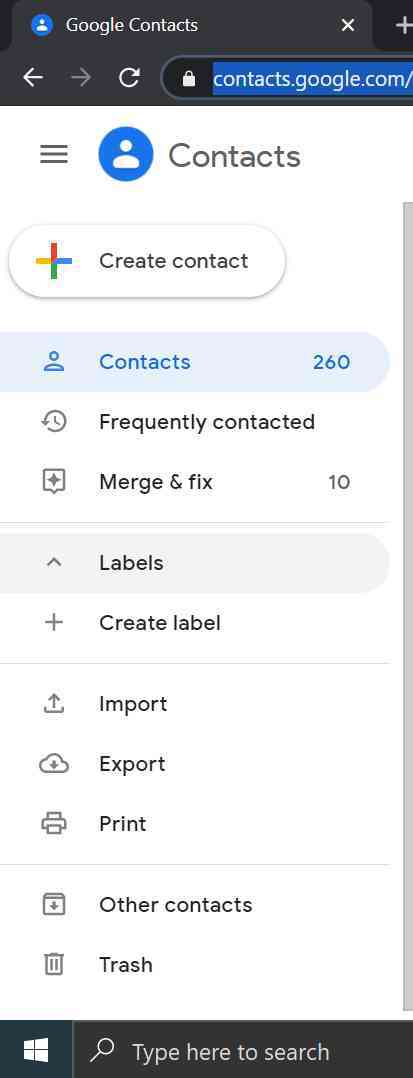This image is a detailed screenshot of a section of the Google Contacts webpage. The main body of the page is white, framed by dark grey bars at the top and bottom. 

In the top left corner, a small blue circle features a white silhouette of a person. Adjacent to this, the text "Google Contacts" is prominently displayed. Moving toward the top right corner, there are options to close the page (an 'X') and add new contacts (a '+' symbol).

Beneath this header, the navigation elements include a left arrow (currently highlighted), a right arrow, a refresh symbol, and a navigation bar featuring a padlock icon followed by a truncated URL, "contacts.google.com/".

The primary content section begins with three horizontal parallel lines on the left, followed by another blue circle with a white silhouette of a person, head, and shoulders, next to the text "Contacts". Below this are the main interactive elements starting with a capsule-shaped button in Google colors that says "Create Contact".

The menu options are as follows:

1. **Contacts** (highlighted in blue) with a symbol of a person and a count of 260 contacts.
2. **Frequently Contacted** with a clock symbol.
3. **Merge and Fix** featuring a plus symbol and indicating there are 10 items.
   
Below these, a grey divider line is followed by:

4. **Labels** and an option to create a new label.

Another thin grey line separates the next set of options:

5. **Import** symbolized by an upload icon.
6. **Export** represented by a cloud with a down arrow.
7. **Print** marked by a printer icon.

A final thin grey line divides the following sections:

8. **Other Contacts** with an accompanying icon.
9. **Trash** symbolized by a trash can.

At the very bottom of the image, the Windows Start icon is visible in the bottom left corner beside a search bar with a magnifying glass labeled "Type here to search."